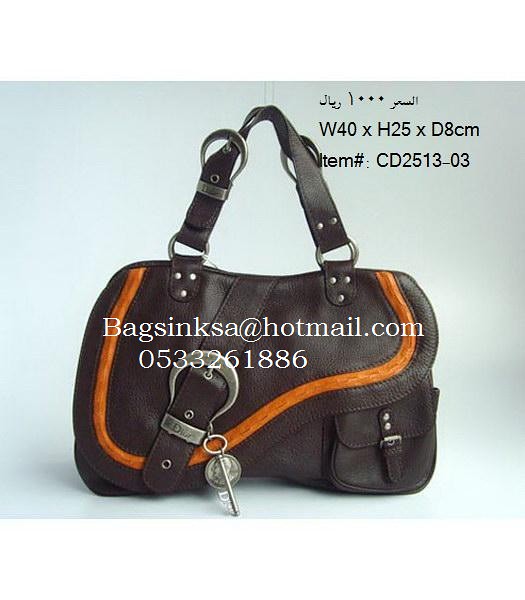This image is a detailed advertisement for a handbag, prominently displayed against a stark white background. The handbag, an elegantly irregularly shaped purse, is primarily constructed from dark brown leather with eye-catching orange striping along its perimeter. The purse features two thick leather straps, adorned with silver hardware, including studs and loops that connect the handles to the bag. The front of the bag showcases a belt-like strap, fastened diagonally with a horseshoe-shaped silver buckle, which holds the bag closed. Attached to this buckle is a charming keychain featuring a skeleton key and a coin charm.

In the top right corner of the image, black text provides the bag’s dimensions (W40 x H25 x D8 cm) and item number (CD2513-03), accompanied by Arabic script. This detail confirms the bag’s compact size. Across the front of the image is a watermark reading "Bags Inksca at hotmail.com 0533261886," indicating the contact information for the seller. The meticulous combination of leather craftsmanship, silver accents, and functional design elements make this handbag both stylish and practical.